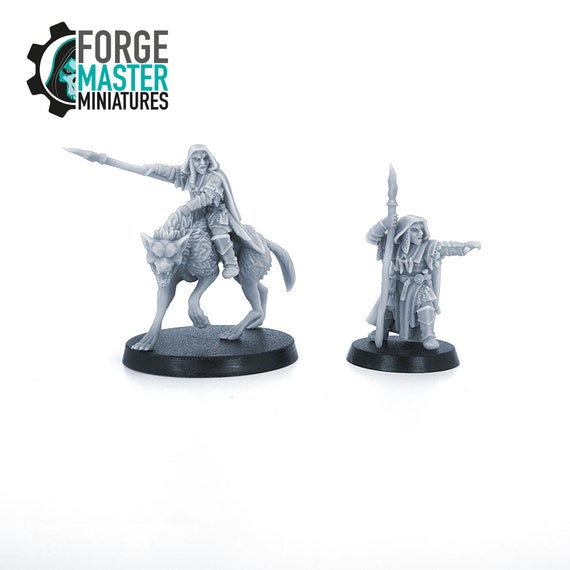This photograph features two highly detailed, uncolored gray figurines from Forge Master Miniatures, positioned on round black bases for display. In the top left corner, the brand’s name is shown in three colors: “Forge” in gray, “Master” in teal, and “Miniatures” in a darker gray, accompanied by a half gear with a skull, likely their logo.

The figurine on the right is a smaller, crouched figure pointing into the distance with his left hand while holding a long, carved stone spear in his right. He is adorned in elaborately detailed, magical fantasy armor with a cloak, belt, long-sleeved tunic, and tall boots.

The larger figurine on the left depicts the same character, who resembles a dwarf or gnome, mounted on a dynamic, spiky-furred wolf, charging forward as if into battle. This rider also wields a spear and is attired similarly in a cloak, boots, long-sleeved shirt, and a tunic.

Both figures exhibit exquisite craftsmanship, particularly in the clothing wrinkles and the intricate details of the wolf’s fur.